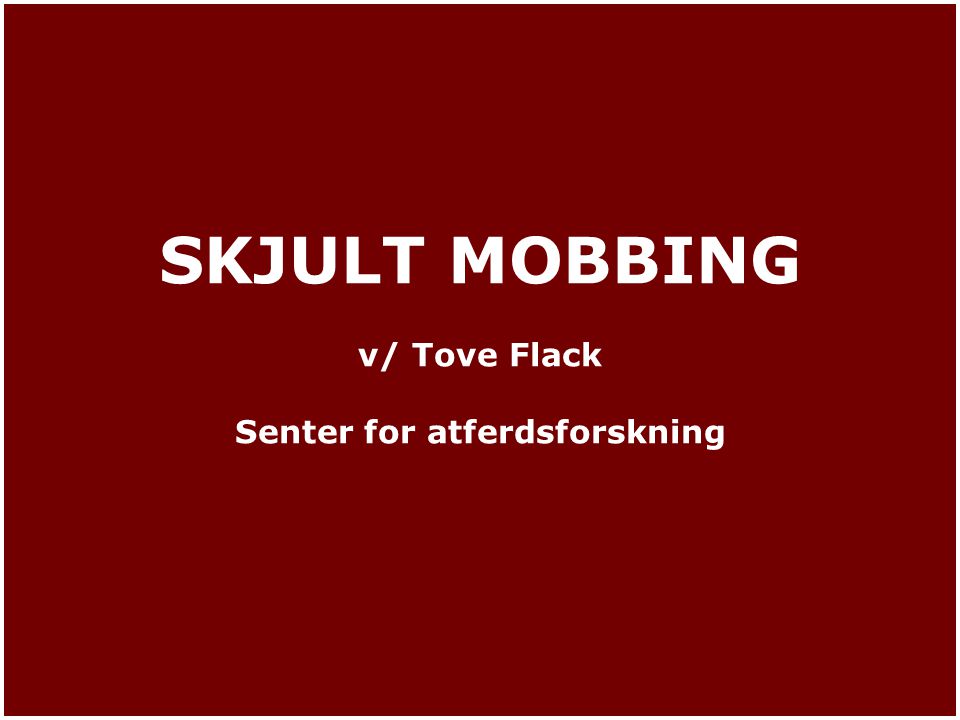The image features a large, dark red rectangle that resembles a deep blood-red or maroon color. Centered within this rectangle is bold white text in large capital letters reading "SKJOLT MOBBING." Directly beneath this, in a smaller font, there is another line of text that says "V/TOV FLACK." Below that, another line of centered text reads, "center for ATF ER DSF OR SK and I NG," with all letters in white, though only the first letter of the final sentence is capitalized. The font throughout the image is sharp and vibrant.